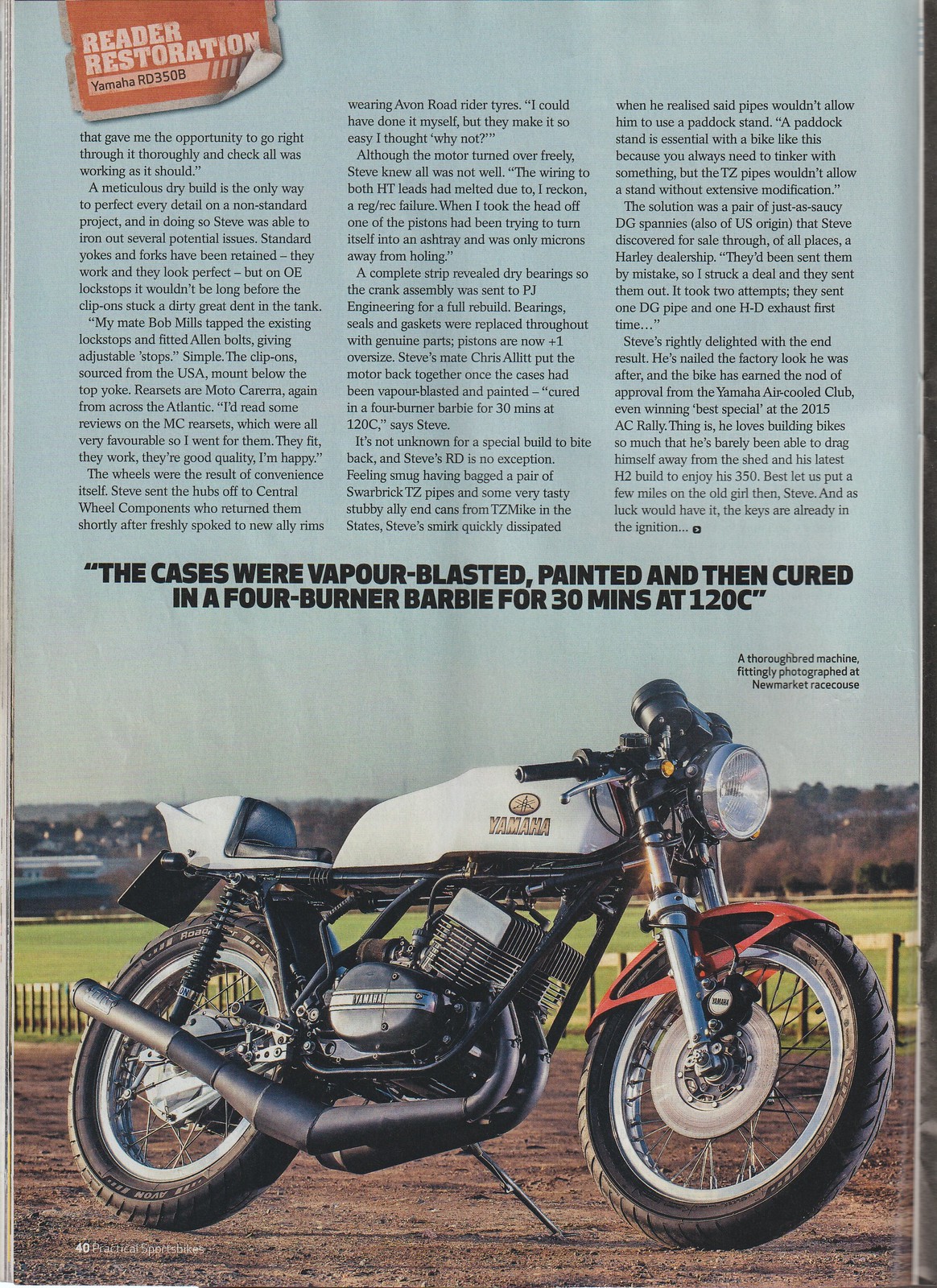The image depicts a photograph of a magazine page, specifically focusing on a motorcycle restoration article. The prominent title at the top reads "Reader Restoration Yamaha RD350B." The middle of the page features an in-depth write-up that includes a notable quote: "The cases were vapor blasted, painted, and then cured in a four-burner Barbie for 30 minutes at 120°C." Central to the image is a Yamaha RD350B motorcycle, distinguished by its white upper section and a red component near the front wheel. The motorcycle, which is shown on a dirt surface with its kickstand down, is captured against a backdrop of grass and a blue sky, adding an outdoor context to the setup. Moreover, the scene's details and impeccable restoration work are highlighted by its setting at the Newmarket Racecourse, emphasizing the motorcycle's quality and thoroughbred status. In the bottom left corner of the page, "40 Practical Sports Bikes" is prominently displayed, suggesting this article is located on page 40 of the magazine.